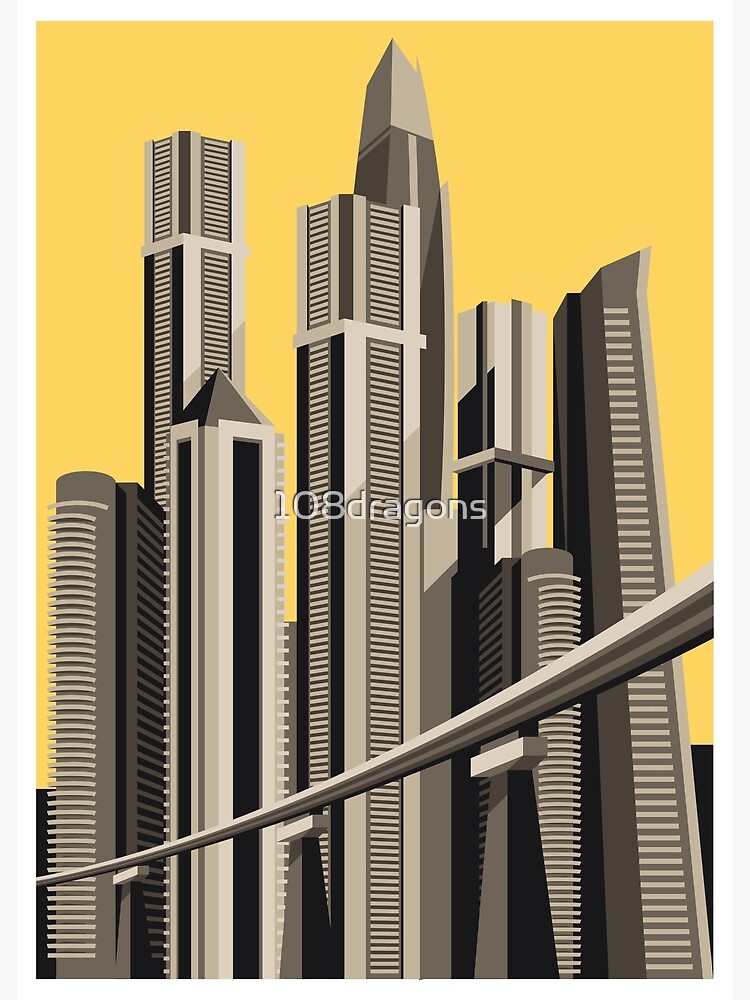The image features an artist's rendition of a futuristic city skyline, rendered in vector art with exceptionally clean lines. Standing out against a golden yellow background, a series of tall, slender skyscrapers—varying in shades of dark gray to light gray and white—dominate the scene. These buildings are characterized by their stylized appearance, with some having sharp, triangular tops while others are flat. They feature rectangular slats that may represent windows. 

The city's skyline includes several main structures: prominently, two extremely tall skyscrapers are situated in the center, with three additional tall buildings on both the left and right sides, forming a dense cluster of high-rising towers. In the foreground, a monorail system stretches left to right, supported by large black triangular columns, hinting at advanced urban transit.

A transparent white watermark in the center of the image reads "108 Dragons," adding a subtle yet noticeable branding to the otherwise sleek and stylized graphic.